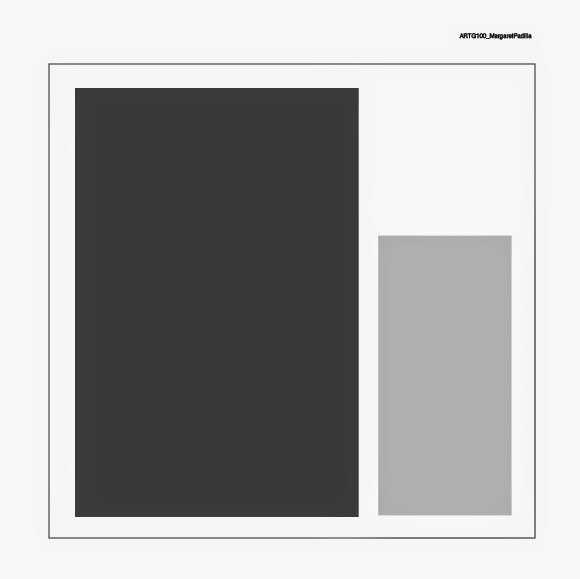This image is a minimalist screenshot from an unspecified source. 

The main structure is a large, white square, within which lies another smaller square outlined in a thin black line. Dominating the interior of this black-outlined square is a vertically oriented black rectangle. Adjacent to this, on its right, is a smaller vertical rectangle in a gray hue. 

In the top right corner of the image, the text "ARTG100_MARGARET_PADILLA" is prominently displayed in uppercase letters.

The image is devoid of any photographic elements, such as people, animals, plants, buildings, bridges, mountains, mechanical objects, or automobiles, emphasizing its stark and abstract nature.